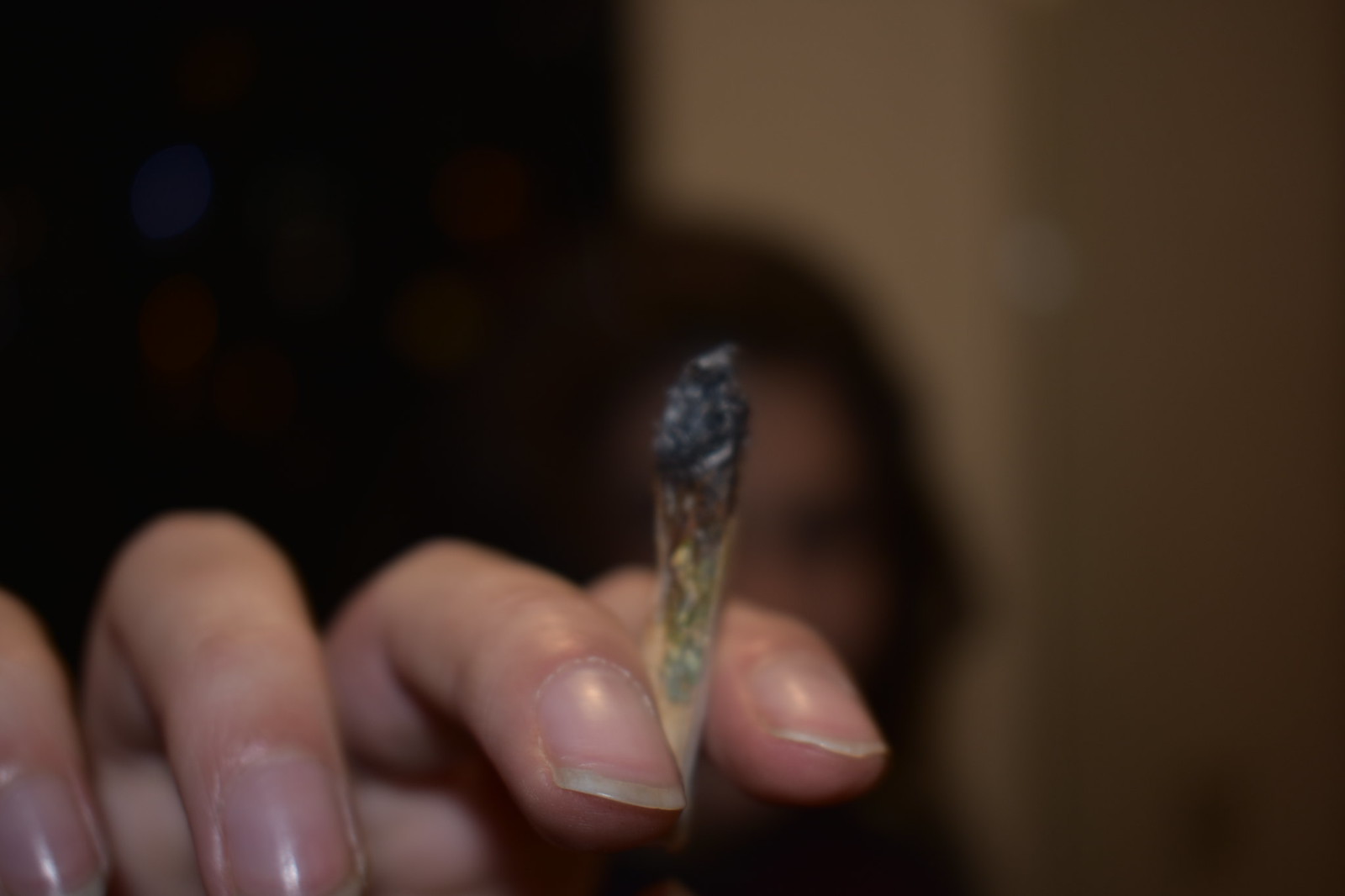The photograph is rectangular in shape and centrally focuses on a Caucasian hand prominently reaching up in front of the camera, holding a marijuana joint, which is burnt about halfway down. The fingers are slightly bent, with rough and jagged fingernails and cuticles, one even appearing a bit dirty. The joint itself transitions from black at the tip to yellowish in the center, with a cream-colored end. The hand is positioned in the lower middle to the left of the image. In the blurred background, there is a silhouette of a woman with long dark hair and feminine facial features, including dark eyes. The surrounding environment appears dimly lit, with colors predominantly being dark brown and black, contrasted by a light tan or possibly white wall. The overall setting seems to be an indoor room.